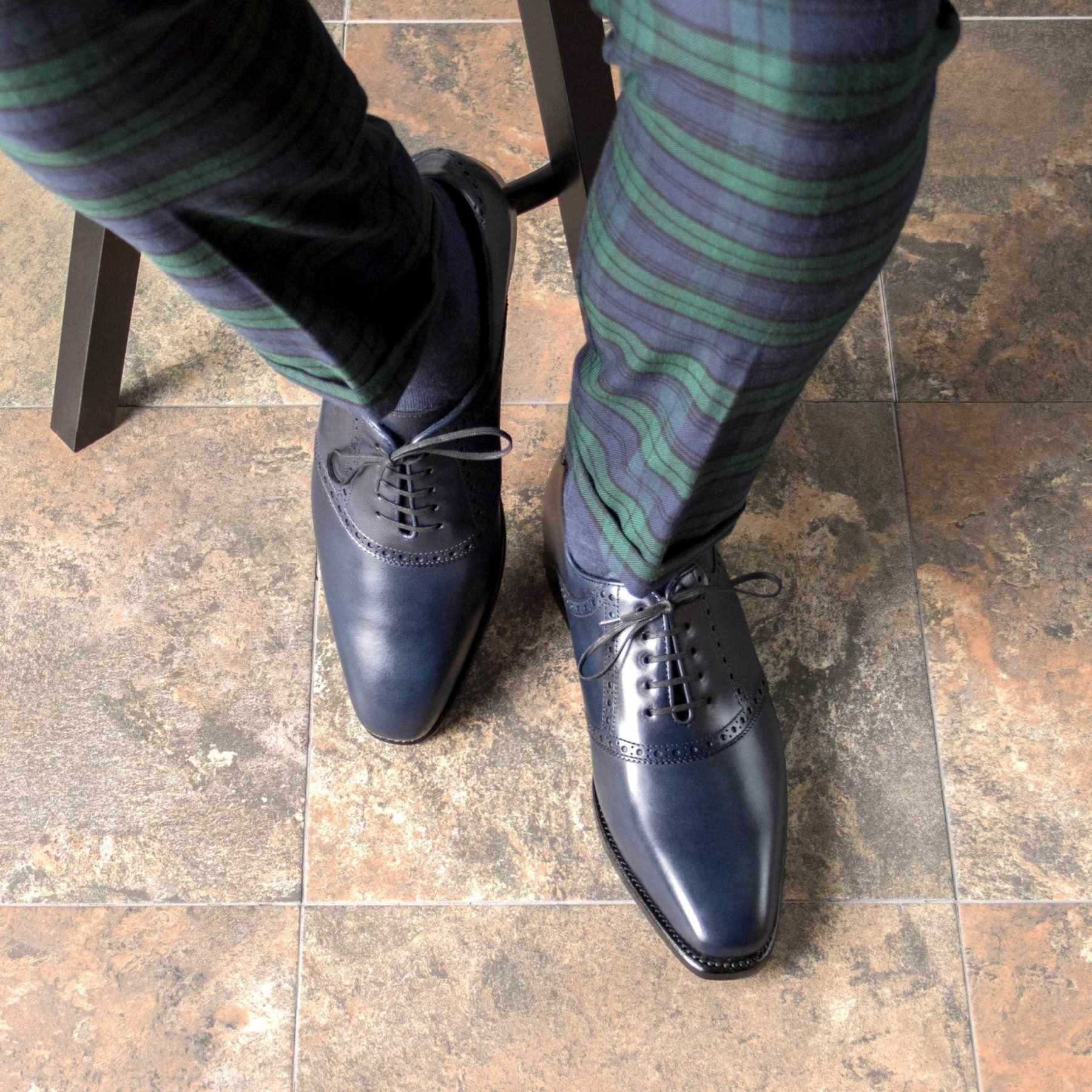This color photograph, oriented in portrait mode, offers a close-up view of a man’s lower legs and shoes, centered primarily around his footwear. The man is seated on a dark brown wooden stool, with his legs extending from the top of the image down to his shoes, which nearly touch the bottom edge. He is wearing green and blue plaid checkered pants that contribute to a semi-casual yet unique aesthetic. His shoes, which are a striking dark blue leather with a polished, shiny finish, have finely detailed stitching around the lace area and feature slim, elegant leather laces that deviate from typical cotton ones, adding a touch of vintage sophistication. One shoe is fully visible and directed towards the viewer, while the other is partially obscured as it is propped against the stool rung. The setting appears to be a kitchen, indicated by the large square tiles on the floor that are a mixture of beige, gray, brown, and pinkish-gray, creating a textured marble effect. The photograph, which adheres to representational realism, captures the fine details of the shoes and the surrounding elements with precision, highlighting the intricate aspects of both the subject's attire and the environment.